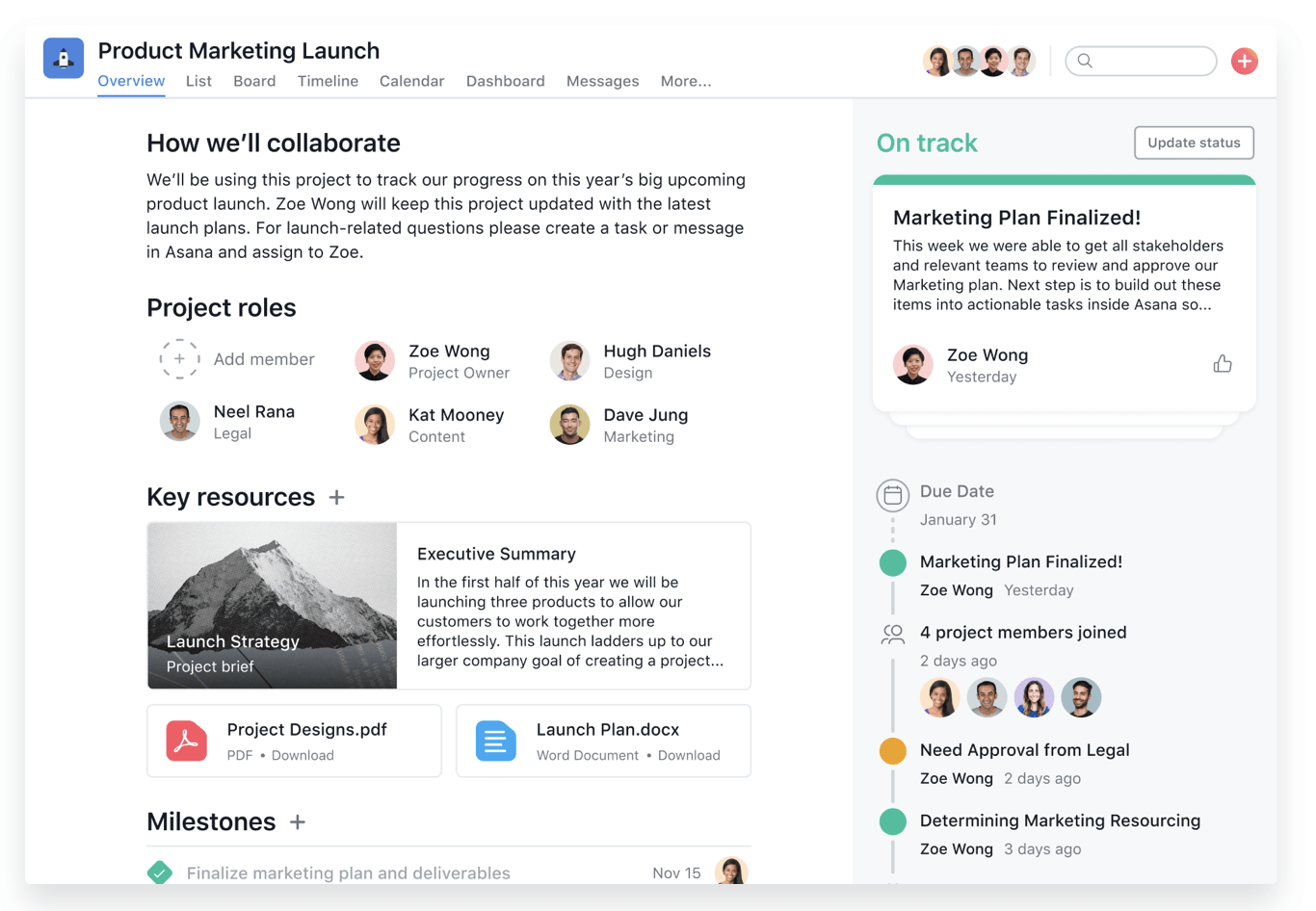This is an image showcasing the overview page of a workplace collaboration software. The design features a clean, white background. In the upper left corner, there's a prominent square purple logo. Adjacent to the logo, the title "Product Marketing Launch" is displayed in bold black letters. Below this title, there is a horizontal navigation bar listing various categories in small grey letters: Overview, List, Board, Timeline, Calendar, Dashboard, Messages, and More. The "Overview" tab is selected, highlighted in blue.

In the top-right section of the page, there are four circular profile pictures arranged horizontally, followed by a search bar. At the far right, there is a noticeable red or yellow circle with a white plus sign inside it.

Just beneath the header, the left side of the page features a bold black heading, "How Will Collaborate," followed by a detailed explanation of the software’s collaborative features. Below that section, another bold black heading reads "Project Roles," listing the participants with their profile pictures to the left, their names to the right, and their specific project roles indicated beside their names.

Towards the lower part of the page, a small grey heading labeled "Key Resources" provides crucial links, including an executive summary, a PDF file for project designs, and a document for the launch plan.

On the left side, the page features a status update section. In the top left of this section, "On Track" is displayed in large green letters. To the right of this status, there’s a white button labeled "Update Status." Below this, there’s a message that reads, "Marketing Plan Finalized," accompanied by a brief description. Underneath the message, the user profile photo and the name of the person who posted it are displayed. Further down the page, there's a vertical timeline segment. At the top of this timeline, the Due Date is noted as January 21st. The timeline also indicates that the "Marketing Plan Finalized" status was updated yesterday.